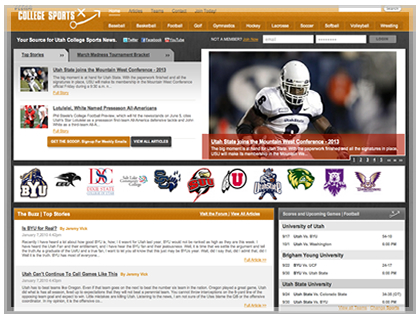The image depicts a sports website dedicated to college sports news, featuring a visually dynamic layout. At the top, a prominent orange banner spans the width of the page. In the upper left corner, the site's name "COLLEGE SPORTS" is displayed in striking white capital letters. Adjacent to the title, a graphic resembling a football play, with an "X," a circle, and an arrow maneuvers around the "X," adds a sporty flair. 

To the top right, there are navigation options: the first highlighted in white and subsequent four in black. At the far right, a white search bar paired with a gray search button invites user interaction. 

Beneath this header, the background shifts to a dark blue or black hue. On the left, white text announces, "Your source for Utah College sports news." Beneath the text, three social media icons—a blue box for Twitter, a blue box for Facebook, and a red box for YouTube—provide quick sharing options. The phrase "Not a member?" is followed by "Join now" in a combination of white and orange text. Below, two input boxes are designated for username and password, next to a gray login button.

Further down on the left, file-tab-like sections alternate between light and dark gray shades. The first tab displays top stories with two highlighted headlines, each accompanied by thumbnail images. One image features a football player in a white jersey, helmet, and shoulder pads cradling a football, with an overlay of a transparent orange banner and white text. The second image appears to show a football player in training gear. Below each headline, long buttons in orange and black with white text offer further interaction.

Below these stories, a horizontal white bar showcases numerous college logos. Familiar logos like BYU, a black bird's head, DSC in red, SUU, and a U with Native American feathers, among others, are lined up. There's also a distinctive green and yellow fur head, a purple and red logo, and a hawk emblem.

At the bottom of the page, additional articles and headlines are interspersed with orange banners for easy visibility. Two headlines, followed by authors' names in orange text, are prominently displayed. To the right, a gray banner lists recent scores, standings, and statistics for universities such as the University of Utah and Brigham Young University, although some other details are not clearly visible.